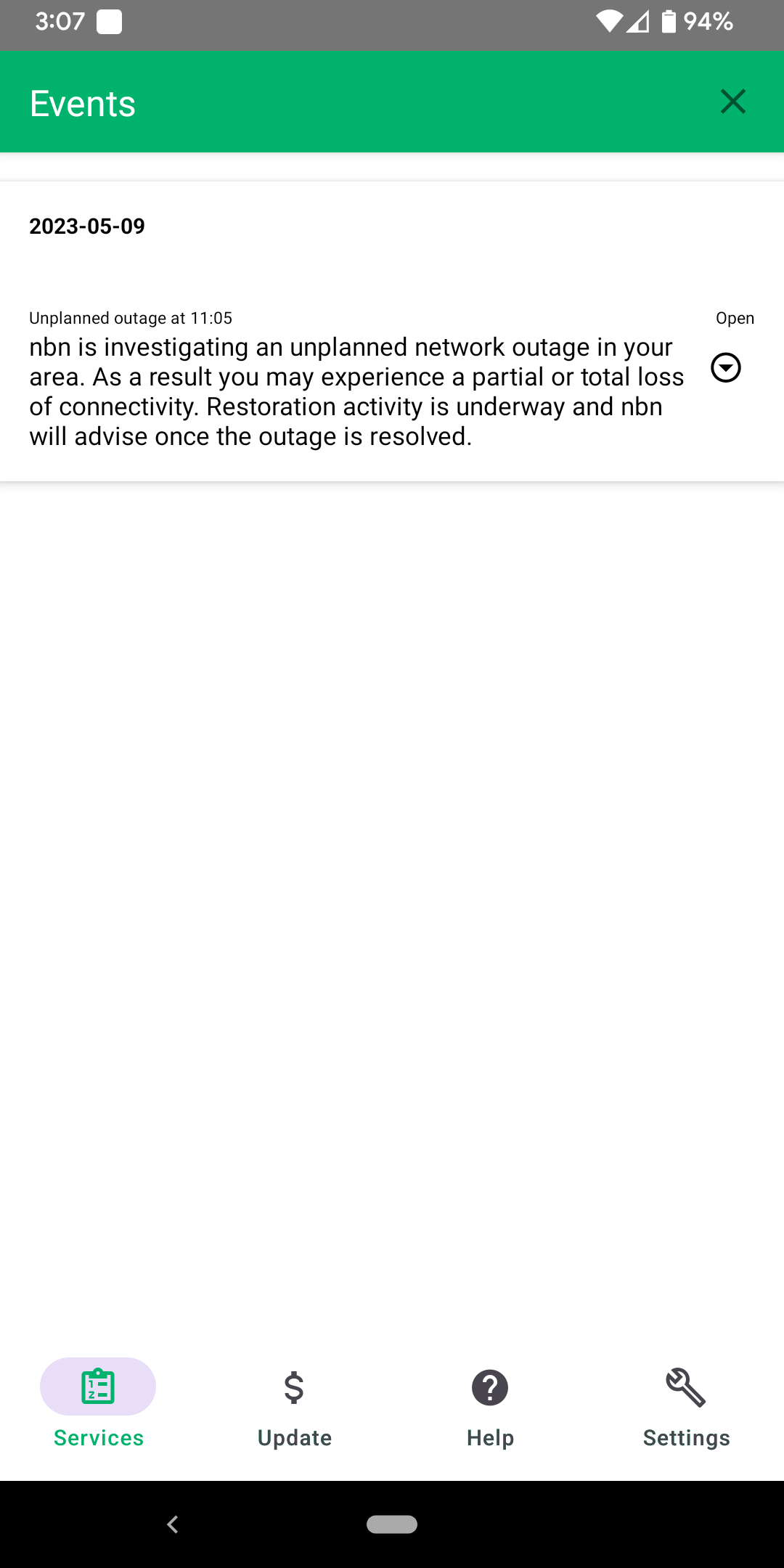A screenshot features a notification interface with a light gray top border. The upper left corner displays the number "307" beside a half-filled signal bar, indicating 94% battery and a full WiFi signal. Just below, a dark green rectangular box is present, with the word "Events" in white on the left side and a black "X" on the right side. A light gray line separates the title from the main content, which begins with black text displaying the date "2023-05-09." 

Beneath the date, a notice reads: "Unplanned outage at 11:05. NBN is investigating an unplanned network outage in your area. As a result, you may experience a partial or total loss of connectivity. Restoration activity is underway and NBN will advise once the outage is resolved." 

Just below this notification, a circular icon with a plus sign inside it bears the label "Open" above. The lower portion of the screen remains largely unused, filled with blank white space. At the very bottom, a green tab labeled "Services" is followed by smaller black tabs for "Update," "Help," and "Settings."